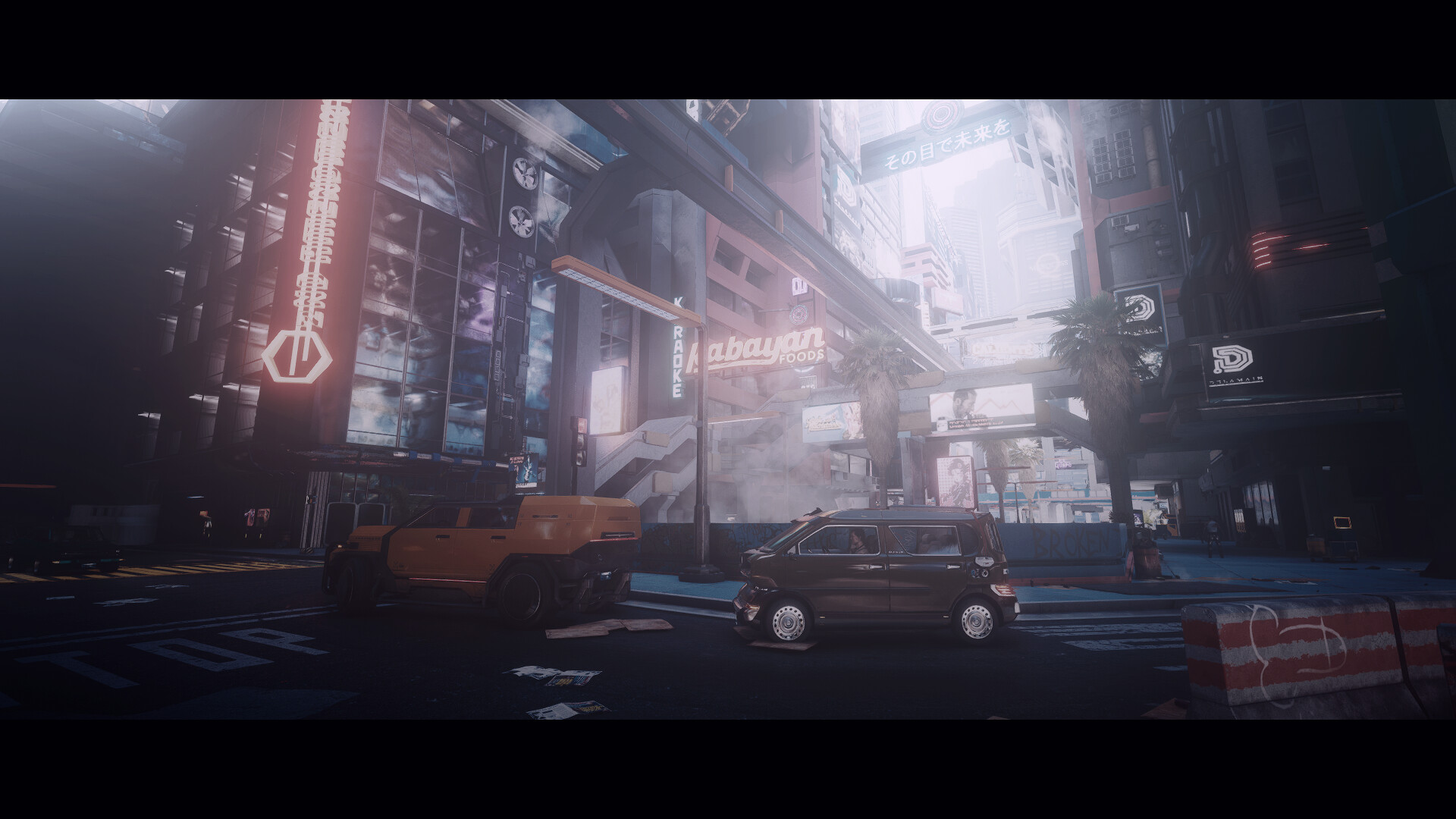The image depicts a digitally generated urban night scene reminiscent of a video game or a photograph of a movie screen. Central to the scene are two vehicles: one is an orange Jeep-like vehicle with black tires, and the other is a small brown SUV, possibly resembling a Morris Minor, also with black tires adorned with silver hubcaps. Both vehicles are positioned on a dark gray road, juxtaposed against a backdrop of towering skyscrapers that dominate the skyline. The buildings are illuminated with various vibrant neon signs, including one in the center that appears to read "Babu Yan," another on the left featuring a pentagon design with vertical text, and a third on the far right which seems to spell out "ID" with illegible smaller text beneath it. Adding an atmospheric touch to the scene, mist or steam rises from the street, and an intense white light emanates from an opening between the buildings. A horizontally striped safety barrier, with prominent orange and gray stripes, is visible in the bottom right corner of the image. The top and bottom of the image are bordered by black, enhancing the cinematic feel akin to watching a film. The overall ambience suggests a desolate, almost abandoned city street, devoid of people, likely set very late at night or in the early hours of the morning.